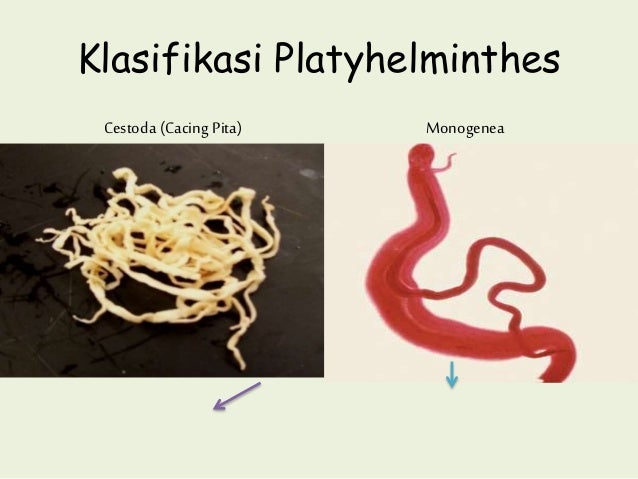The image features a detailed illustration of worm-like organisms against a light gray background. At the top of the image, in black lettering, is the title "Klasifikasi Platyhelminthes." The image is divided into two sections: on the left, there is a rectangular shape with a black background displaying a pile of yellowish, spaghetti-like organisms, possibly Sistota. To the right, there is a drawn red worm-like creature labeled "Monogenea," with a small blue down arrow beneath it. The overall setup resembles a PowerPoint slide intended for educational purposes, displaying a range of colors including light green, black, yellow, red, light blue, and purple.